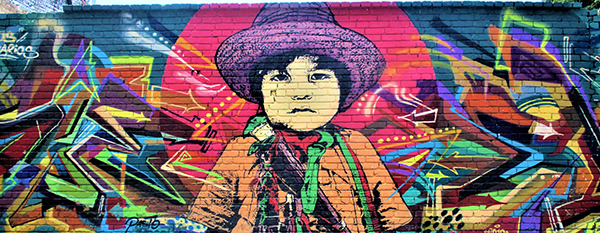This image captures a wide-angle shot of a brick building adorned with a vibrant mural. The focal point of the mural is a serious-looking little boy wearing a purple brim hat and a brown jacket, adorned with a mix of colorful sashes or ties in hues like green, purple, and red. His face is notably yellow. He stands prominently against a teal blue background, with a distinct hot pink circle right behind him. Surrounding the boy are multicolored arrows and lightning bolt-like designs, adding dynamic energy to the piece. The mural is rich with vibrant colors such as green, yellow, purple, red, and orange, making the entire wall a canvas full of life. In the upper left-hand corner of the mural is some lettering, possibly the artist's signature. Additionally, the building on which this mural is painted stands before another white brick building, glimpsed in the upper left-hand corner of the image.